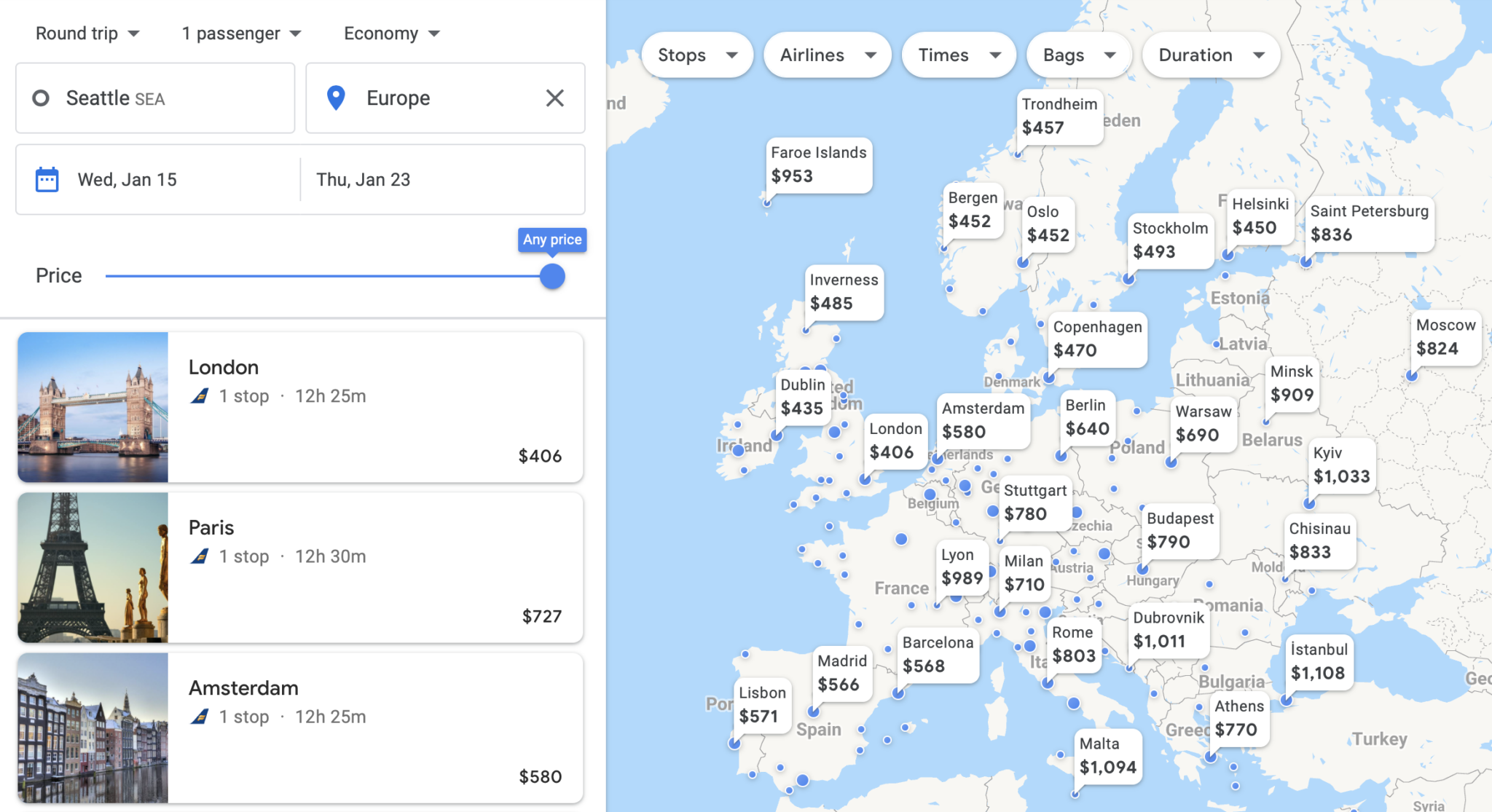This horizontal image, likely captured from a smartphone or computer screen, presents a clean, white background typically associated with digital interfaces. In the upper left corner, options are displayed for booking a flight, with selections highlighted for a round-trip, one passenger, and economy class. The departing location is Seattle, with a European destination for the travel period of Wednesday, January 15th through Thursday, January 23rd.

The search results list flight options to three European cities—London, Paris, and Amsterdam—detailing the number of stops, travel duration, and prices. Flights to London are shown as having one stop, lasting 12 hours and 25 minutes, priced at $406. Flights to Paris involve one stop, 12 hours and 30 minutes in duration, priced at $727. Flights to Amsterdam, with one stop, last 12 hours and 25 minutes, and are priced at $580.

On the right side of the image, a map is displayed, accompanied by filters for stops, airlines, times, bags, and duration. Cities are listed alongside their respective flight prices, all presented in a white box with black font for clear readability.